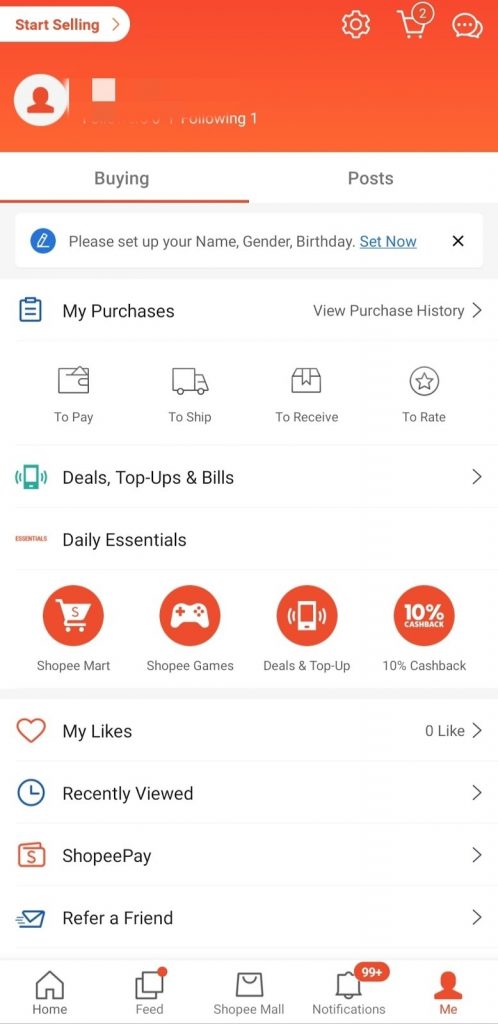At the very top of the image, the background is a bright orange, complemented by a white circle containing a profile image of a person. Above this, in another white circle, there is the text "Start Selling." Below the profile photo, in gray text underlined in orange, is the word "Buying."

Moving down, there is a blue circle featuring a pencil icon, accompanied by the text "Please set up your name, gender, birthday," and then in blue text underlined, "Set Now." Beneath this section, there is an image of a notebook next to the words "My Purchases," with the option "View Purchase History" to the right.

Further down, various options are listed in a row: "To Pay," "To Ship," "To Receive," and "To Rate." Below this row, there is an image of a green cell phone with three options: "Deals," "Top-Ups," and "Bills."

Next, there is an orange circle with a shopping cart icon and the label "Shopee Mart." There are similar orange circles with icons and labels such as "Shopee Games" (video game controller), "Deals and Top-Up" (cell phone), and "10% Cashback."

The final section lists choices in a vertical order: "My Likes," "Recently Viewed," "Shopee Pay," and "Refer a Friend." At the very bottom right corner, in orange, is the word "Me."